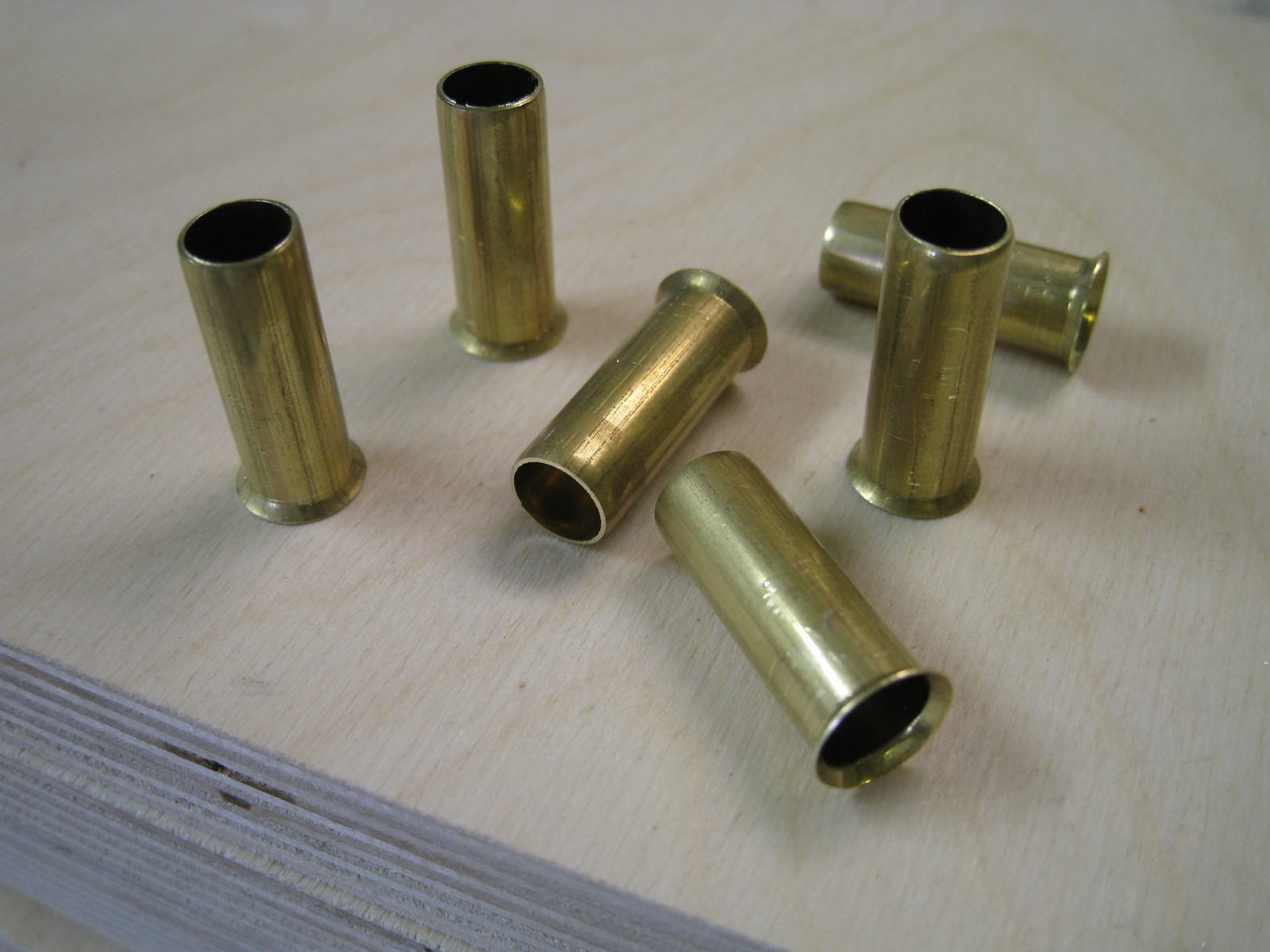The photograph captures six brass-colored cylinder-shaped objects, resembling empty shell casings, arranged on a thick, light wooden surface that showcases its grainy texture prominently. The surface occupies most of the image, with the bottom left revealing its grainier edge, suggesting a well-sanded, sturdy wooden desk or table. Three shell casings are standing upright: two are positioned on the left and one on the right. Between the two on the left, a shell lays flat with its top facing down and to the left. To the right of the standing shell, another lies flat with its top pointing up and to the left. In the bottom right foreground, the last shell lays flat with its top also pointing up and to the left, mirroring the positioning of the one in the middle. All shell casings have small black holes at their tops and cast noticeable shadows on the wooden surface. A subtle bluish tint is visible along the side of the desk or table, adding a slight color variation to the composition.